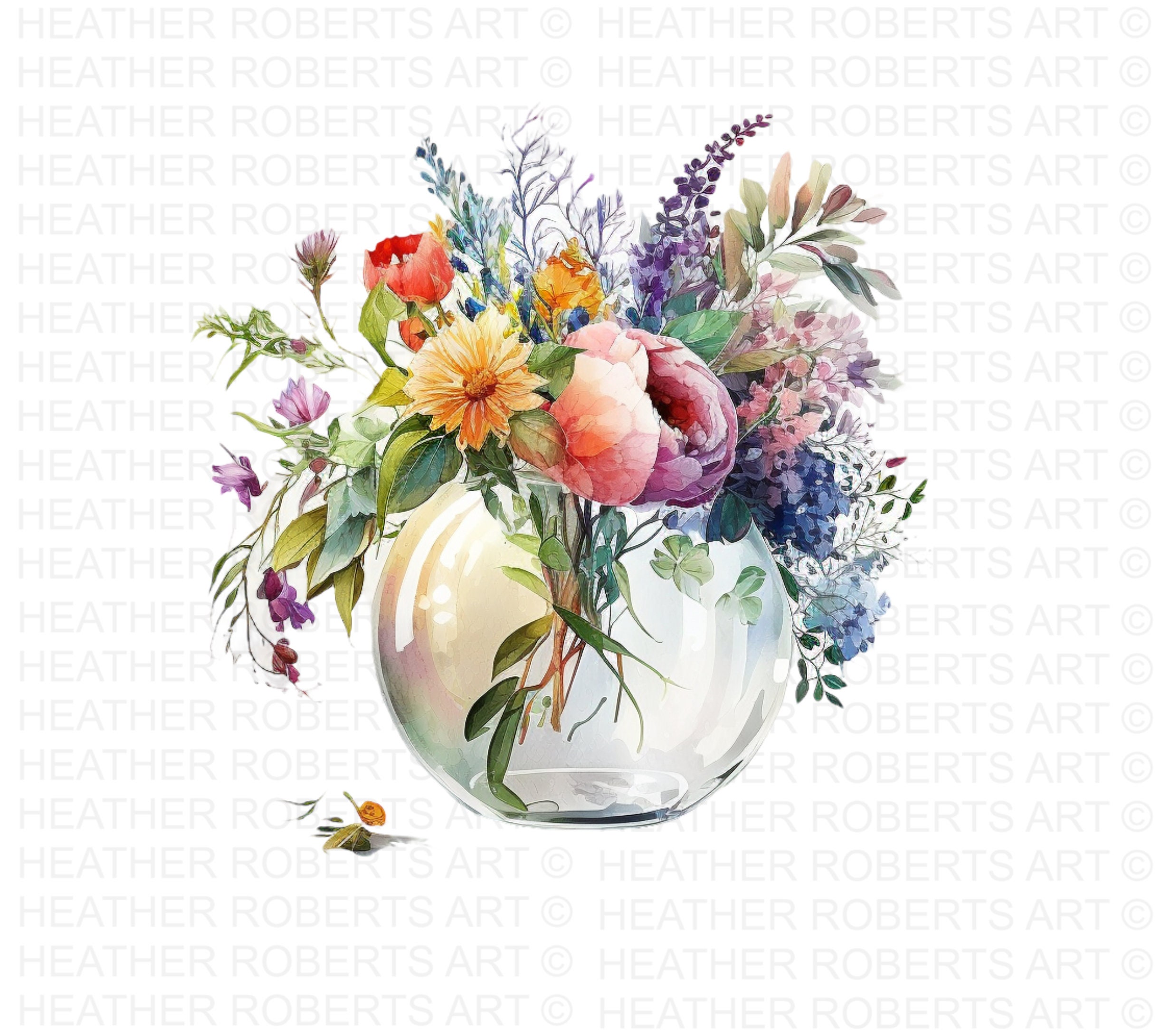This detailed descriptive caption is a synthesis of the three provided captions, emphasizing shared and repeated details:

This artwork is a graphic design or hand-drawn realistic painting of a large, bold vase filled with a variety of flowers. The arrangement features an array of vibrant colors, including pink, orange, purple, red, and blue. Notably, there is a pointed flower with yellow-tinted petals on the center left, and a uniquely round flower that appears half-purple and half-pink on the right. The flowers are housed in an oval-shaped glass bowl, reminiscent of a fishbowl, which is filled with water. Below the floral display, some leaves have fallen off one of the plants and rest on the bottom left of the bowl. In the background, a watermark that reads "Heather Roberts Art" is subtly repeated throughout, covering the entire image with the text. This repetitive watermark ensures the attribution to Heather Roberts Art is unmistakable.